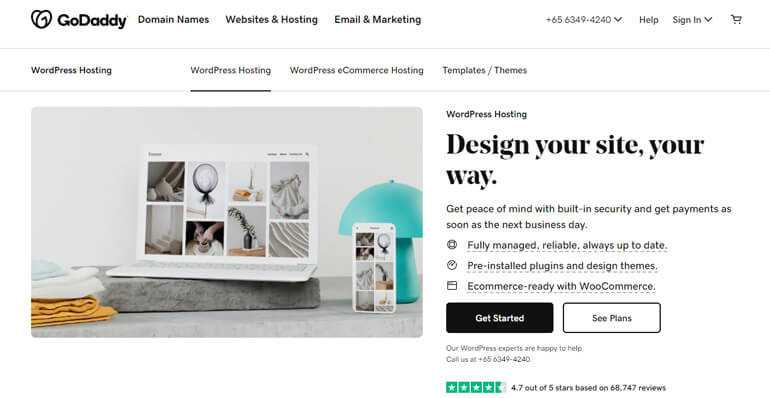This is a detailed description of a website page:

The screenshot shows a web page with a clean, white background and a structured layout. At the very top, there's a header. On the left side of this header, there's a bold black title reading "GoDaddy." To the right of this title, in smaller black text, are the categories: "Domain Names," "Websites & Hosting," and "Email & Marketing."

Towards the top-right corner of the header, you see grey text displaying a phone number: "+65 6349 4240," accompanied by a downward-facing arrow. Further right, you find "Help" and "Sign In," each with their respective downward arrows indicating drop-down menus. Next to these, a shopping cart icon is displayed. Below this header, a thin, light grey line runs across the width of the page, demarcating the header from the content below.

The next section of the page is another header. On the left, in small black text, it says "WordPress Hosting." To the right, the section is divided into three similarly styled links: "WordPress Hosting" (underlined in black), "WordPress eCommerce Hosting," and "Templates/Themes." Another thin light grey line runs beneath this menu.

The body content of the page starts beneath this line, maintaining the white background. The layout is predominantly divided into a left two-thirds section featuring a photograph and a right one-third section containing text. The photograph has a horizontal rectangular shape with rounded corners, showcasing a marble countertop. On this countertop, there's a stone slab with a white laptop placed on it. The laptop screen displays images of various household objects. To the left of the laptop, there's a neatly stacked set of towels. To the right, there's a blue lamp with a mushroom shape, along with a white smartphone leaning against it. The smartphone screen mirrors the display of household objects seen on the laptop.

On the right side of the page, there’s large, bold black text that says "Design Your Site Your Way." Above this title, it reads "WordPress Hosting" in smaller text. Below the title, there's a line of small black sans serif text that states, "Get peace of mind with built-in security and get payments as soon as the next business day."